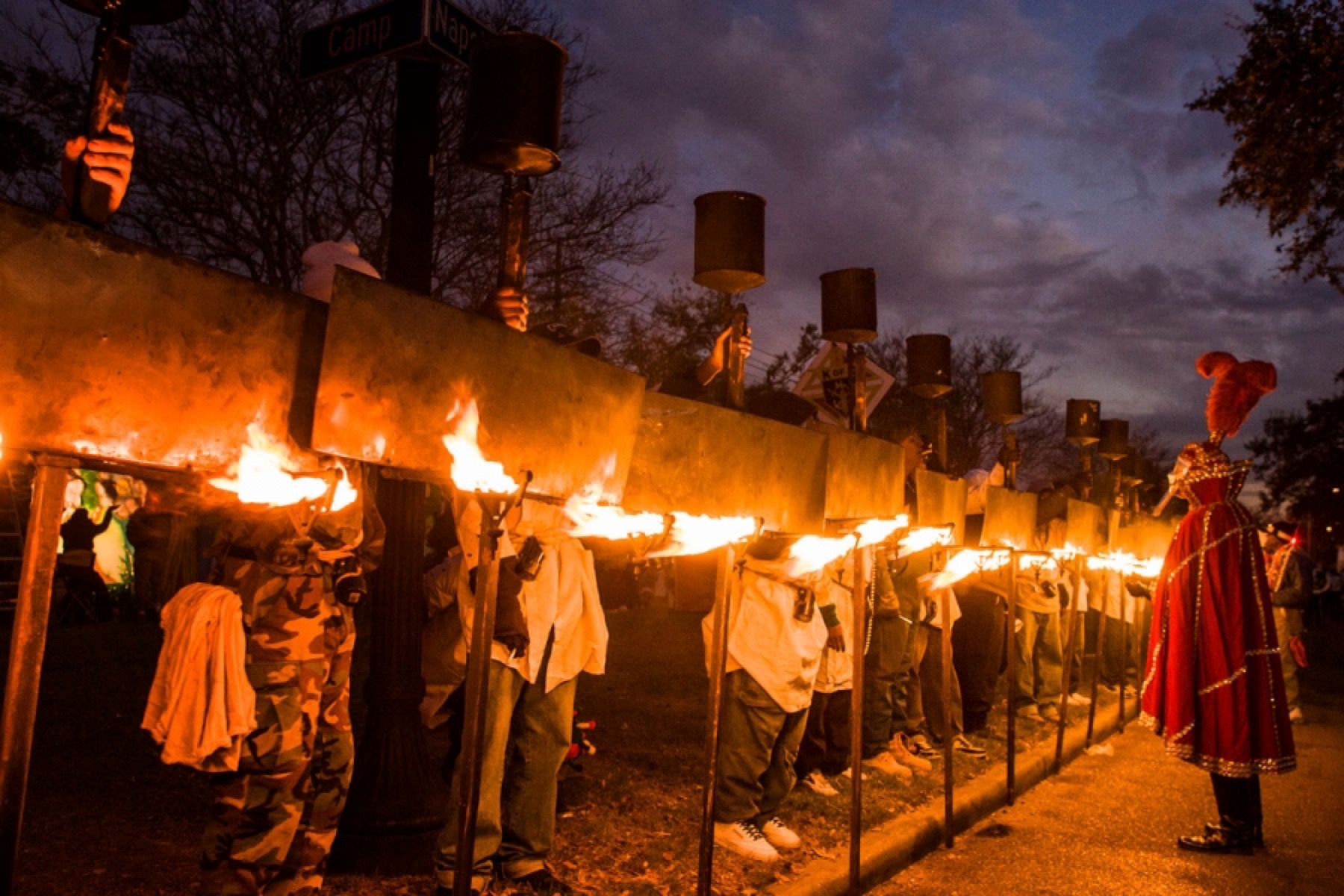The photograph captures a nighttime traditional ritual set against a dark, cloudy, and purple-hued sky with trees in the background. A central paved road is bordered by grass and a narrow drain. The scene is populated by participants in various traditional costumes. Dominating the right side, a man is dressed in an elaborate costume with a large silver opera mask featuring an elongated nose, a gray wig, and adorned with two red feather plumes. He sports a red high-collar cloak with gold trim that partially hides the back of his head and tall leather knee-high boots.

In front of him, arranged along a curved line, multiple wooden staves with torches are planted, each bearing large metal plaques. The torches are alight, adding an atmospheric glow to the scene. Holding each stave is a person dressed in traditional clothing, mostly white kurtas with grey trousers and sneakers, and one individual in an armed forces camouflage uniform. The man in the center is distinguished by his red gown with golden sequins and petal designs, black pants, and shoes. His headgear, which includes the large red feathers, matches the elaborate costume of the man on the right, emphasizing the ceremonial and traditional nature of the event.